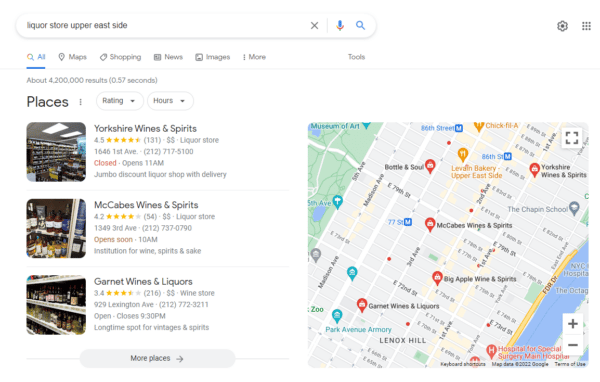**Detailed Caption of the Image:**

The image displays a search results page from an online suggestion bar focused on a liquor store on the Upper East Side. The selection is highlighted in blue under the "All" tab, with additional tabs for Maps, Shopping, News, Images, and More shown adjacent to it. Centered on the page, there's a toolbar where these tabs are displayed prominently.

Below the toolbar, the search results are listed, starting with:
1. **Yorkshire Wines and Spirits**: The store's name is followed by its address and a note that it opens at 11 a.m. It is described as a "Jumbo Discount Liquor Shop with delivery," accompanied by a photograph of the store's interior.
2. **McCabe's Wine and Spirits**: Accompanied by a picture focusing on wine bottles arranged on a rack, this store is described as an institution for wine, spirits, and sake. The address is also provided.
3. **Garnet Wines and Liquors**: This listing includes a photograph of a wine shelf and mentions the store's long-standing reputation for vintages and spirits. The address is listed as well.

A clickable option to "See more places" is available for those seeking additional locations.

On the right side of the page, a map of Manhattan is shown with red pins marking seven different locations where one can purchase wine and spirits on the Upper East Side.